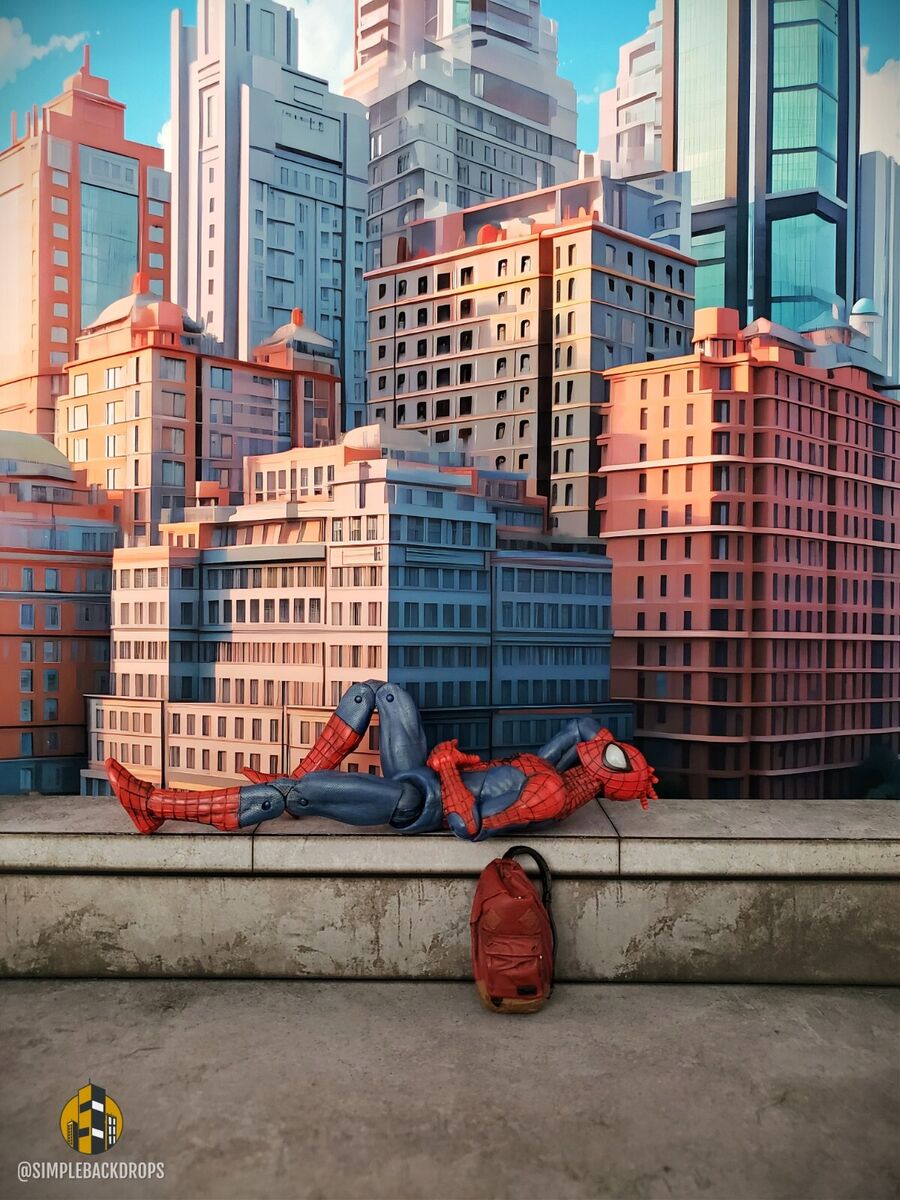This image appears to be a CGI-enhanced photograph featuring a Spider-Man action figure posed on a grey concrete ledge. Spider-Man, dressed in his iconic red and blue suit with a full mask, is lying in a relaxed position: his right knee is bent upwards, his right hand rests behind his head, and his left arm lies across his torso. Adjacent to him lies a narrow, brown backpack standing against the ledge.

The background showcases a detailed New York City skyline with buildings of varying heights and colors. The buildings closest to Spider-Man are predominantly brownstones, intermixed with some of blue and white hues. As the cityscape extends, skyscrapers appear in blues, reds, and occasional greens. Notably, one building features a small dome, which could signify a notable city structure such as a city hall. The image has a label at the bottom reading "Simple Backdrops."

The overall composition highlights both the leisurely pose of the Spider-Man figure and the intricate cityscape, blending elements of digital art and photography for a compelling visual effect.